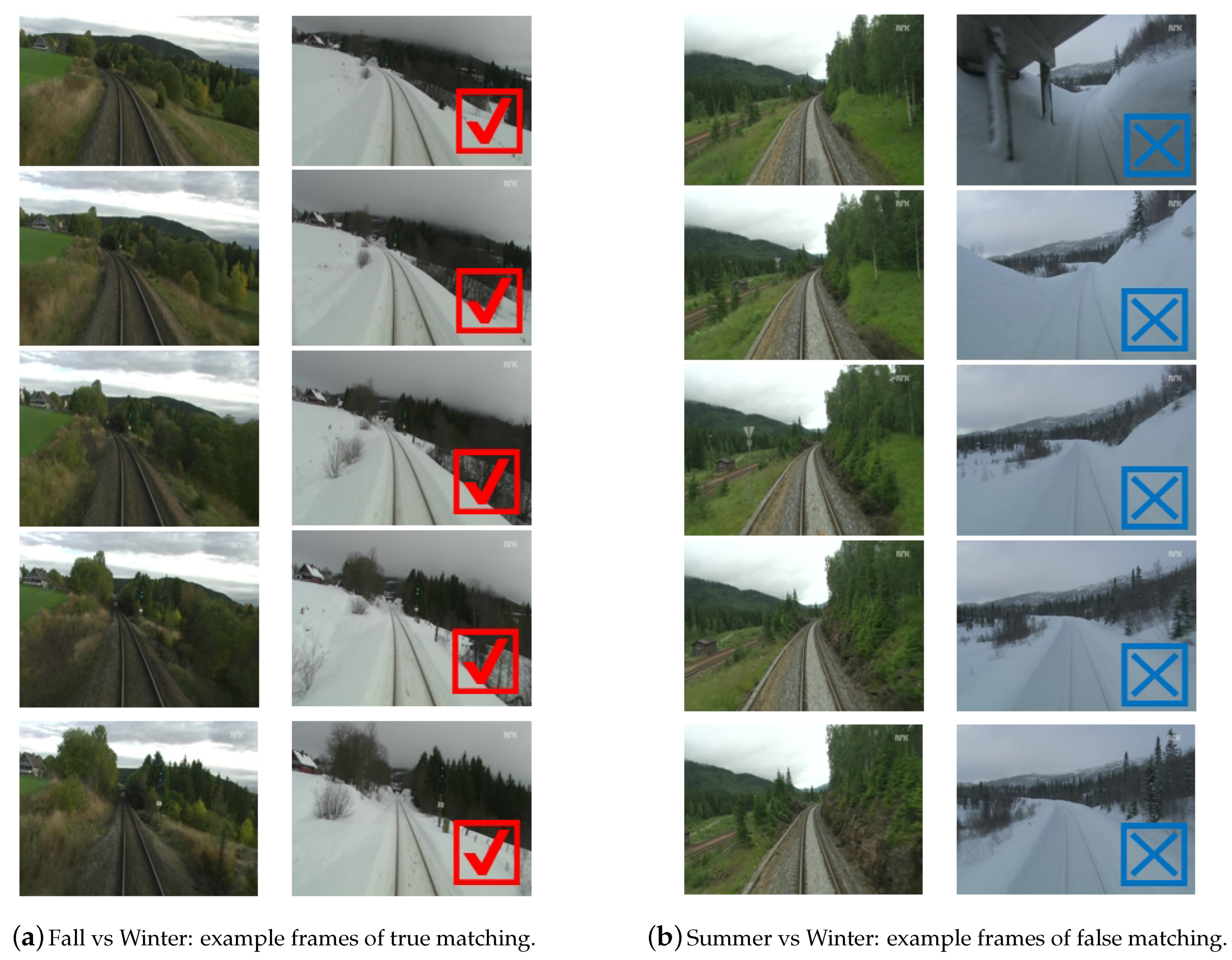This image features a comparative analysis of seasonal transformations in a landscape, specifically highlighting railroad tracks. It is divided into two sections, A and B, each containing ten photos arranged in four vertical columns. Section A, labeled "Fall vs. Winter: Example Frames of True Matching," consists of the first two columns. The left column displays five images of train tracks winding through lush, green forests on a cloudy day, indicative of fall. The adjacent right column depicts the same locations under winter conditions, where the forests are blanketed in snow. Each photo in the winter column bears a red check mark at the bottom right corner, indicating true matching.

Section B, titled "Summer vs. Winter: Example Frames of False Matching," occupies the last two columns. The left column shows five images of train tracks cutting through green mountain terrain on a cloudy summer day. In contrast, the right column presents images of snowy landscapes with train tracks, but these do not correspond to the same locations as their summer counterparts. These winter images feature a blue box with a blue X in the bottom right corner, signifying false matching. Each photo set illustrates the seasonal differences and their impact on terrain recognition, emphasizing true versus false matches. A faint watermark appears in the upper right-hand corner of the screen, though the text is illegible.